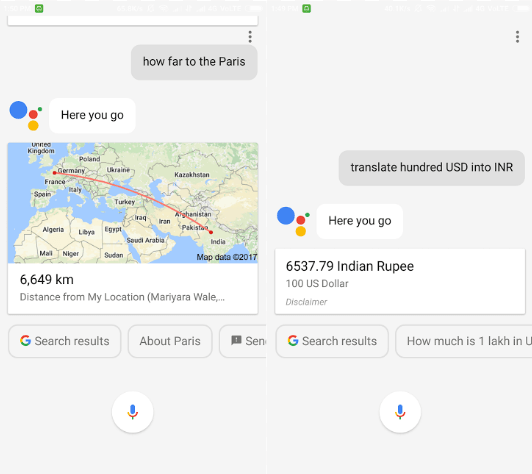**Detailed Caption:**

The image displays a Google search interface featuring an AI-powered response. At the top, there is a gray background text bubble with the user’s search query, "How far to Paris?" The query appears to activate a response from an AI, indicated by the multicolored Google dots. The AI responds with "Here you go," followed by a map beneath the text.

The map is a small rectangular section showing a vast geographical area from the United Kingdom to India, including parts of Africa. A prominent red line on the map marks a route from a starting point in India to Paris, France. The indicated distance is 6,649 kilometers.

Below this, another search query is displayed, "Translate 100 USD into INR," to which the AI also responds with "Here you go," followed by the conversion result: 6,337.79 Indian Rupees. This further solidifies the presence of Google's AI handling and generating responses for the user's inquiries.